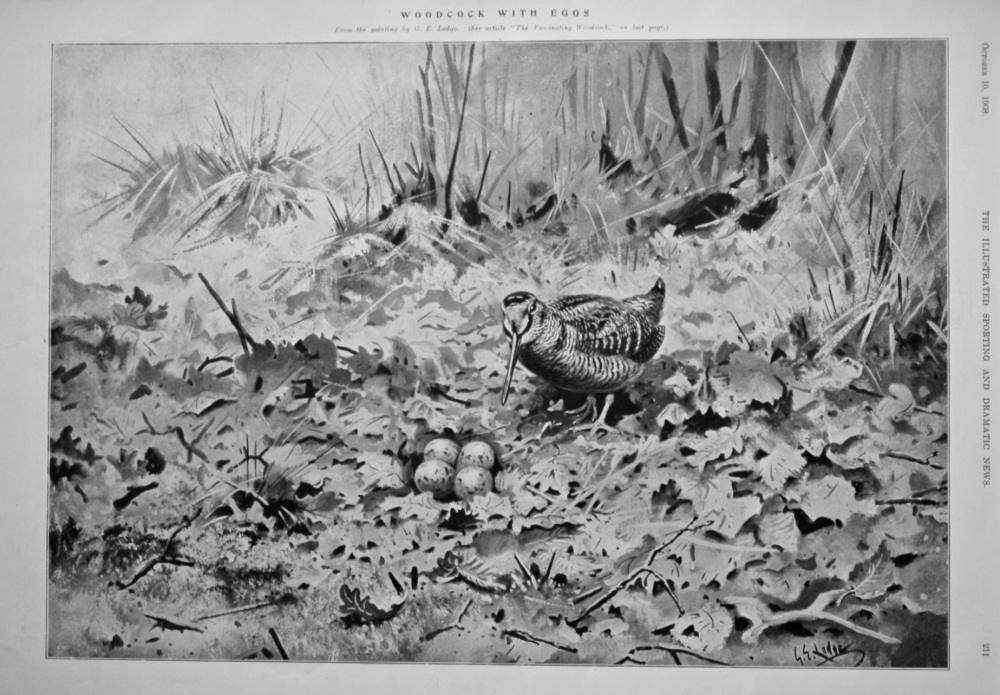This black-and-white artwork depicts a nature scene featuring a bird, identified as a woodcock, standing on the ground amidst leaves and tall blades of grass. The bird, positioned slightly right of center, showcases distinctive black and white striped feathers and a notably long beak. The bird appears to be tending to four speckled eggs nestled among the leaves. The intricate drawing captures the forest floor's detailed textures, including twigs and grass blades, which create a dense background. At the top of the piece, the title "Woodcock with Eggs" is clearly inscribed. The right-hand side of the image features the vertical text "The Illustrated Sporting and Dramatic News," which may indicate the source or publisher. In the bottom right corner, there is an artist’s signature, rendered scribbly and in black, alongside the figures "2-1-1," which may serve as an identifier or catalog reference. The small text beneath the title remains illegible.